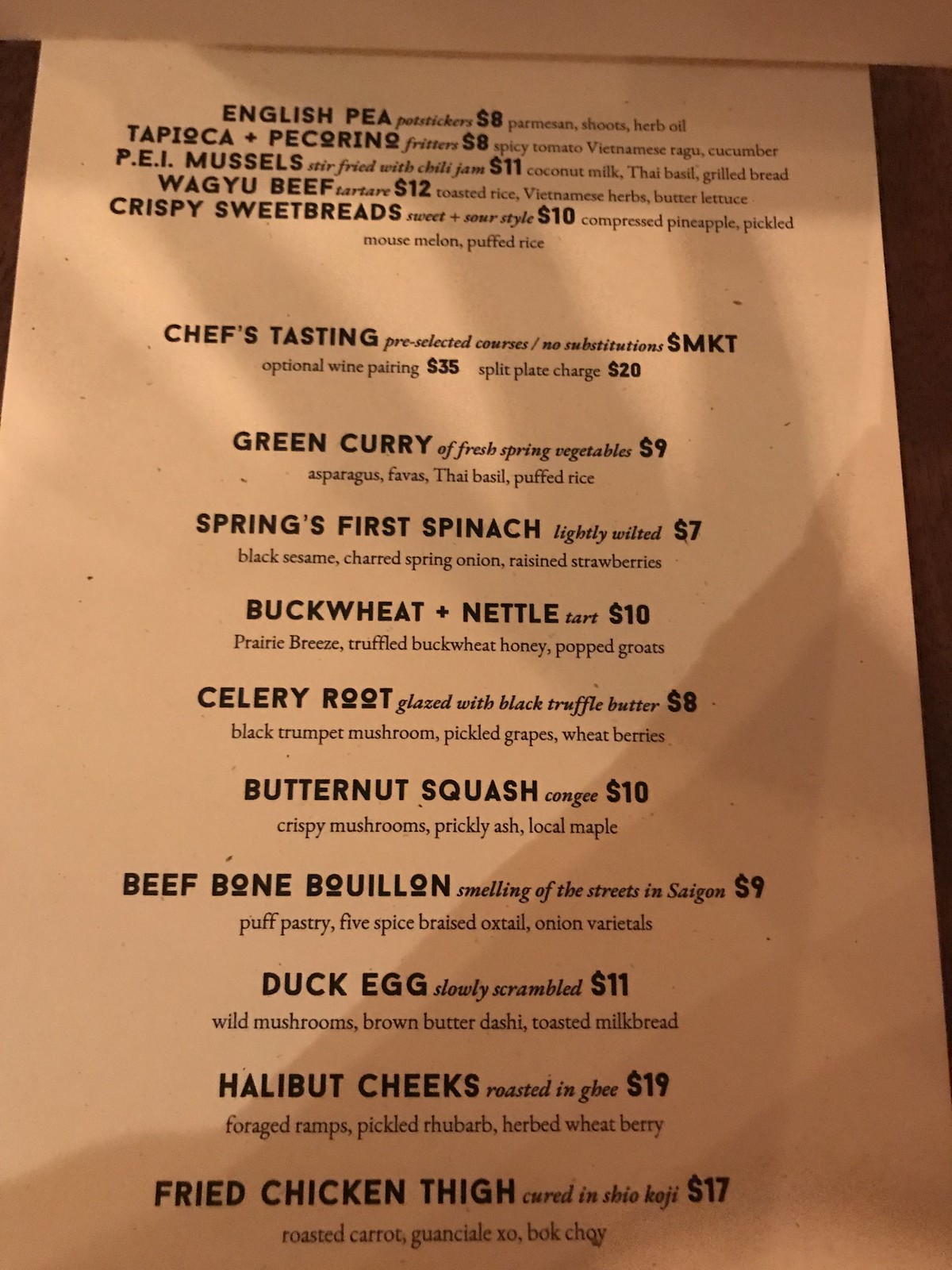**Detailed Caption:**

The image displays a restaurant menu printed on white paper with black typeface, where certain elements are emphasized in bold. The names of various soups and dishes, along with their prices in American dollars, are featured prominently. Notable shadows are visible on the paper, particularly concentrated in the lower left and right corners, extending upwards and across the left corner. The shadows reveal the distinct outline of four fingers towards the upper right portion of the menu, suggesting someone is holding the menu during the photograph.

The menu begins with "English Pea Potsticker" priced at $8, characterized by Parmesan shoots, herb oil, and tapioca and pecano fritters. Another item is the "Spicy Tomato Vietnamese Ragu" listed at $8, which includes cucumber and PEI mussels stir-fried with chili clam jam. Following this is a dish of "Coconut Milk Thai Basil Grilled Bread Wagyu Beef Tartare" costing $12, featuring toasted rice, Vietnamese herbs, and butter lettuce.

"Sweetbreads, Sweet and Sour Style" priced at $10, comes with compressed pineapple, pickled mouse melon, and puffed rice. There is also a "Chef's Tasting Menu" with preselected courses, available at market price, with an optional wine pairing for $35. A split plate charge of $20 is also mentioned.

For vegetarian options, "Green Curry of Fresh Spring Vegetables" is listed at $9, comprising asparagus, fava beans, Thai basil, and puffed rice. Additionally, the menu includes "Spring's First Spinach" which consists of buckwheat and nettle, celery root, butternut squash, beef bouillon, duck egg, slowly scrambled, and halibut cheeks roasted in ghee, paired with a fried chicken thigh.

This detailed menu, partially obscured by shadows and fingers, provides a glimpse into the sophisticated offerings of the restaurant.